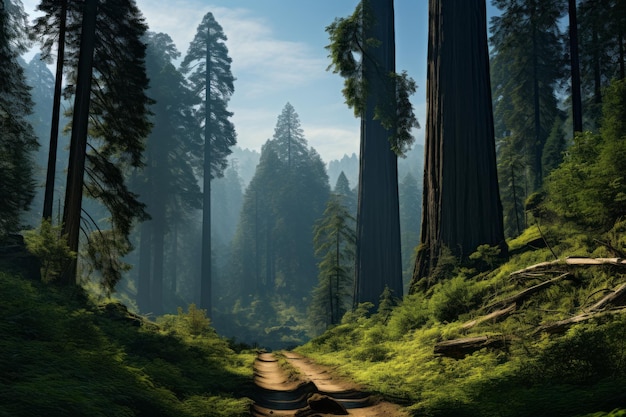In this hazy color photograph of a forest, a brown, dusty trail—resembling a two-lane dirt road—winds through the scene, leading into the depths of a dark and densely forested area. The foreground features a lush, mossy green grass that transitions into a blur as the perspective deepens. Tall trees with brown trunks dominate the landscape, their leaves clustering only at the tops, silhouetted against the hazy mid-ground. The forest floor is scattered with bits of bark, branches, and fallen leaves. On the right-hand side, thick silhouetted tree bases stand starkly against the softer background. Further in, there's a large tree surrounded by multiple smaller ones, all fading into various shades of light and dark, hinting at more vegetation veiled in mist. The sky peeks through the V-shaped canopy in the upper center of the image, showcasing patches of blue dotted with puffy white clouds, suggesting a beautiful day despite the haze enveloping the trees.